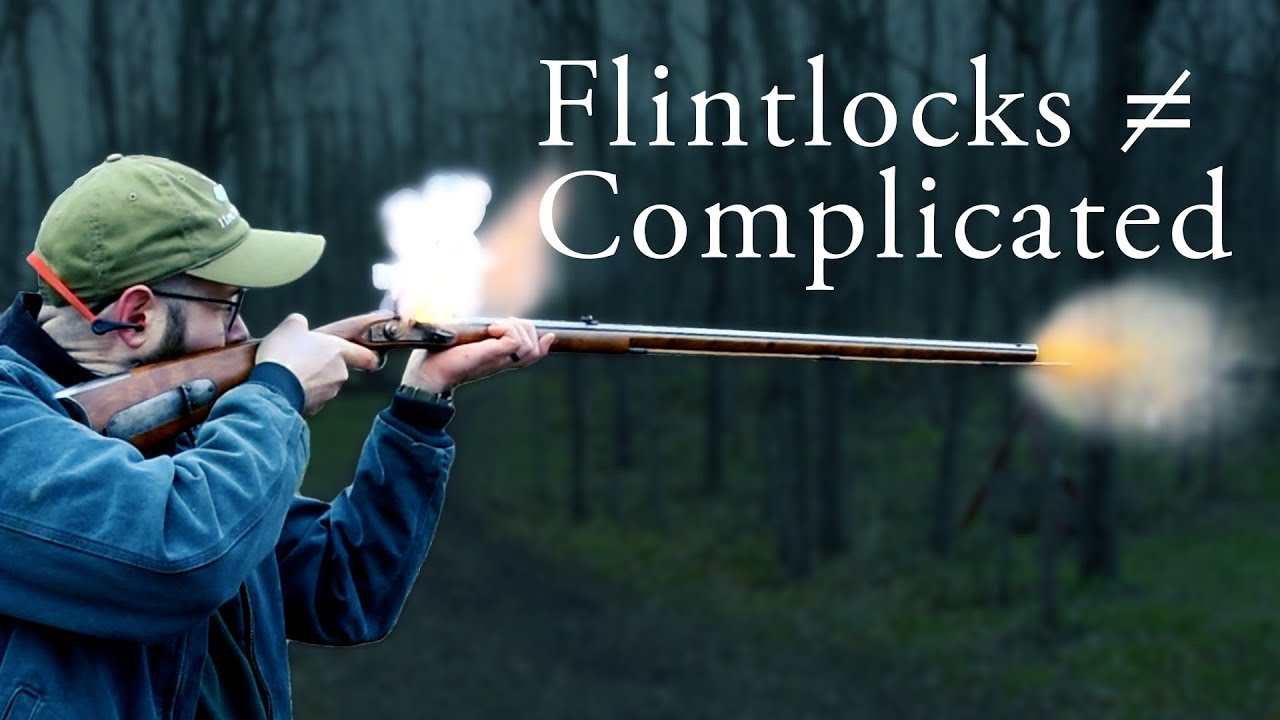The photograph is a YouTube thumbnail featuring a man firing a rifle amidst an out-of-focus woodland backdrop. White text in a complex font reads "Flintlocks ≠ Complicated." The man, positioned on the left side of the image, wears an olive green hat, protective black earmuffs with an orange strap across the back, black eyeglasses, and a blue denim jacket. A vivid muzzle flash is visible at the end of his brown wooden-stocked rifle with iron sights, and smoke clouds emerge from both the muzzle and the handle, indicating the gun has just been fired.